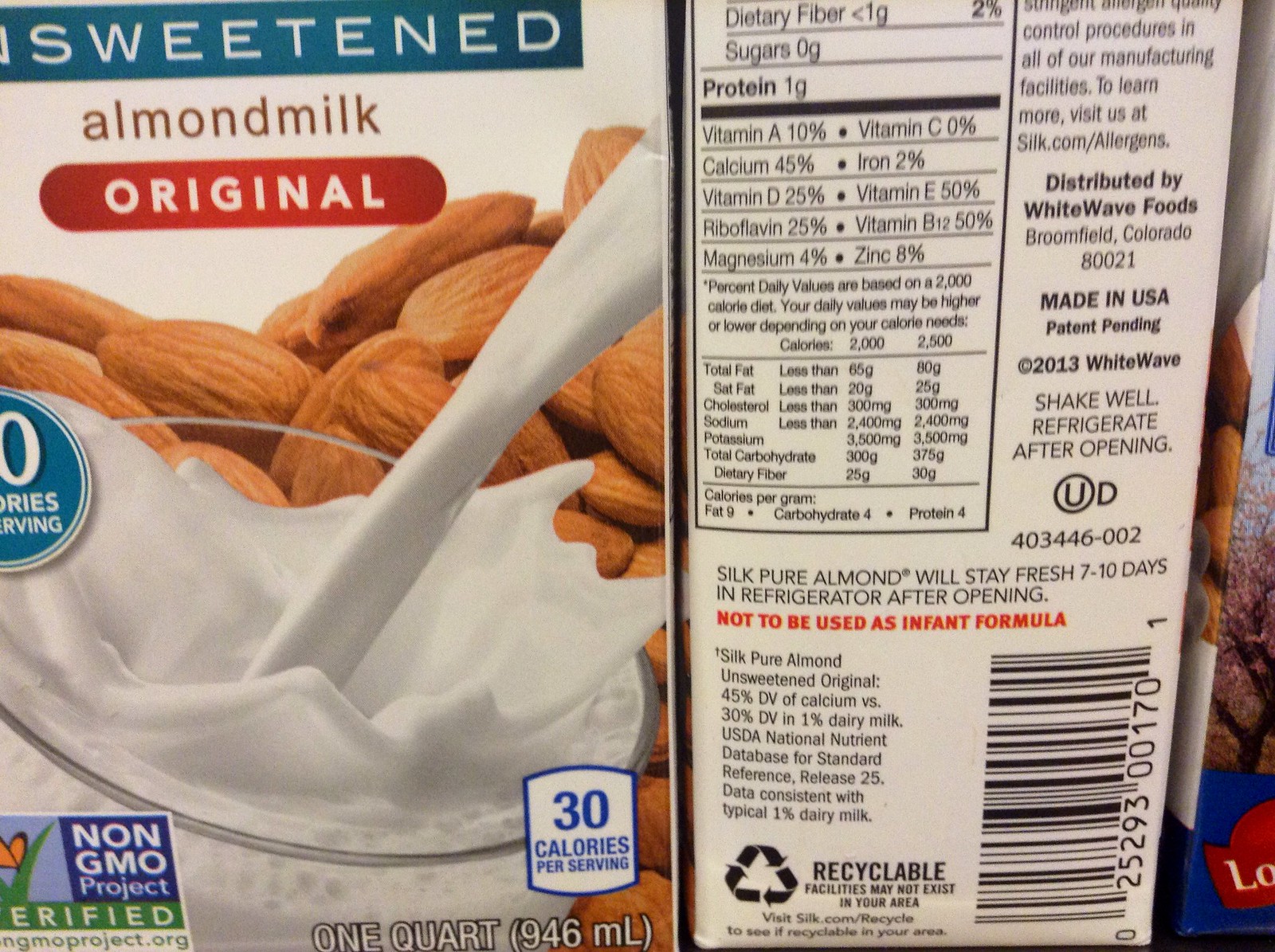The image is a color photograph featuring two cartons of almond milk. The carton on the left shows the majority of its front-facing label, which reads "Unsweetened Almond Milk Original." The label includes a photographic illustration of raw almonds alongside milk being poured into a clear glass, artfully splashing up from the rim. The text at the bottom left indicates it is "Non-GMO Project Verified," and the bottom right mentions "30 calories per serving," with a volume of "1 quart" or "946 milliliters." The carton on the right is turned sideways, displaying its nutritional information and other details. The visible nutritional facts include less than one gram of dietary fiber, zero grams of sugars, and one gram of protein, along with various vitamins and minerals. Additional text notes that the product is distributed by White Wave Foods, based in Broomfield, Colorado, USA, with a patent pending from the year 2013. Instructions advise to "Shake Well" and "Refrigerate After Opening," with the milk remaining fresh for 7 to 10 days post-opening. A clear warning in bold red letters states, "Not to be used as infant formula." Other symbols include a UPC code, a kosher certification, and a recyclability disclaimer suggesting facilities may not be available in all areas.